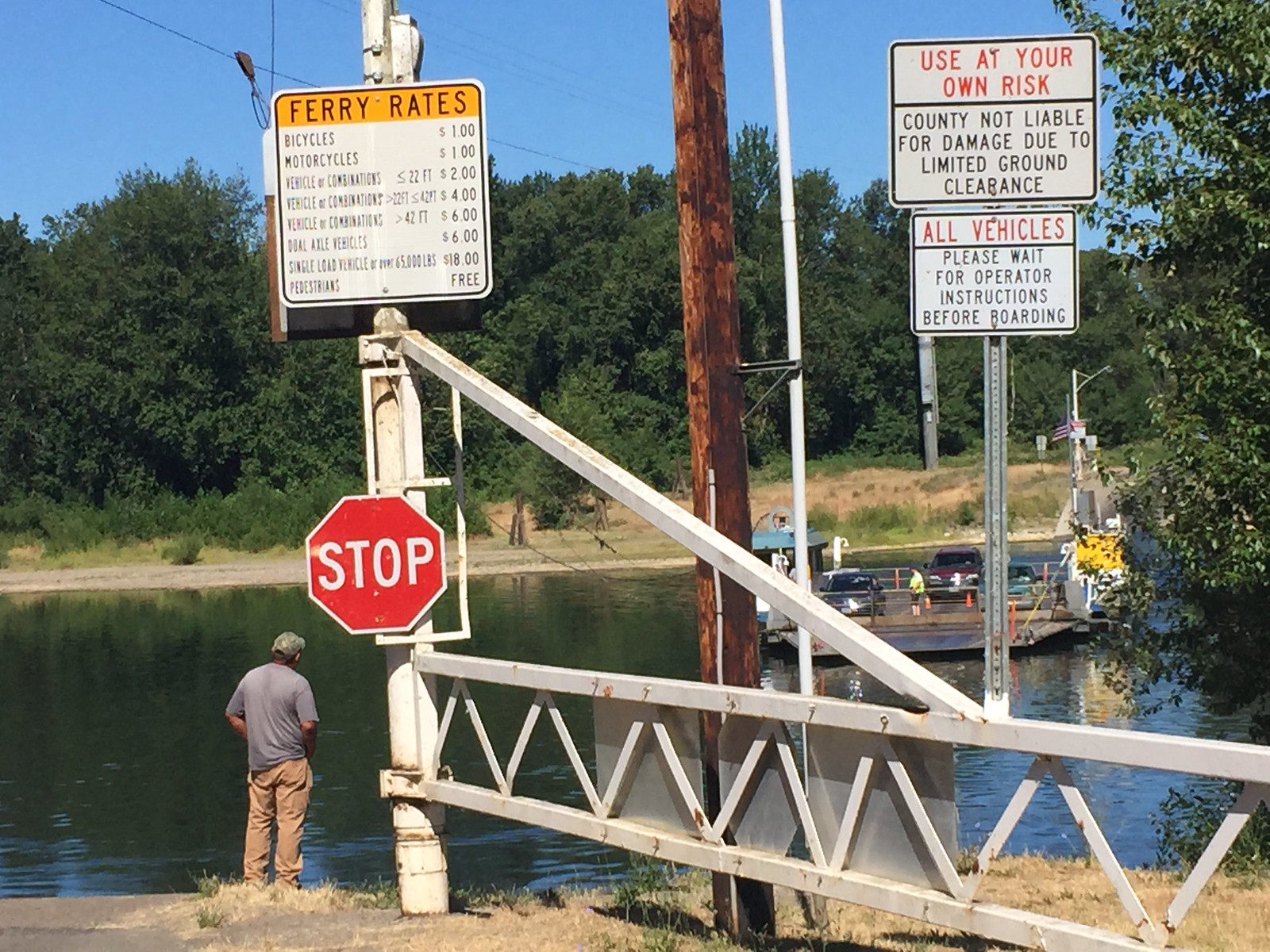The photograph captures a detailed scene at a ferry dock, set against a picturesque lake or river. In the foreground, a white metal gate stands open, with a red stop sign attached on the left of center. Above the gate, a white sign with a yellow stripe lists the ferry rates, including bicycles and motorcycles for $1, various vehicles for $2, $4, $6, up to $18, and noting that pedestrians cross for free. A man, standing on the lower left corner beside the gate, wears beige/tan pants, a blue/gray t-shirt, and a baseball cap, gazing across the water. The land appears dry, with patches of dry grass near the dock. Further on the dock, another sign advises, "Use at your own risk, County not liable for damage due to limited ground clearance," and instructs vehicles to wait for operator instructions before boarding. The ferry itself, visible to the right of the image, carries about three cars and a few people, making its way across the green waters. Trees frame the opposite shore, adding to the serene yet functional atmosphere of the scene.